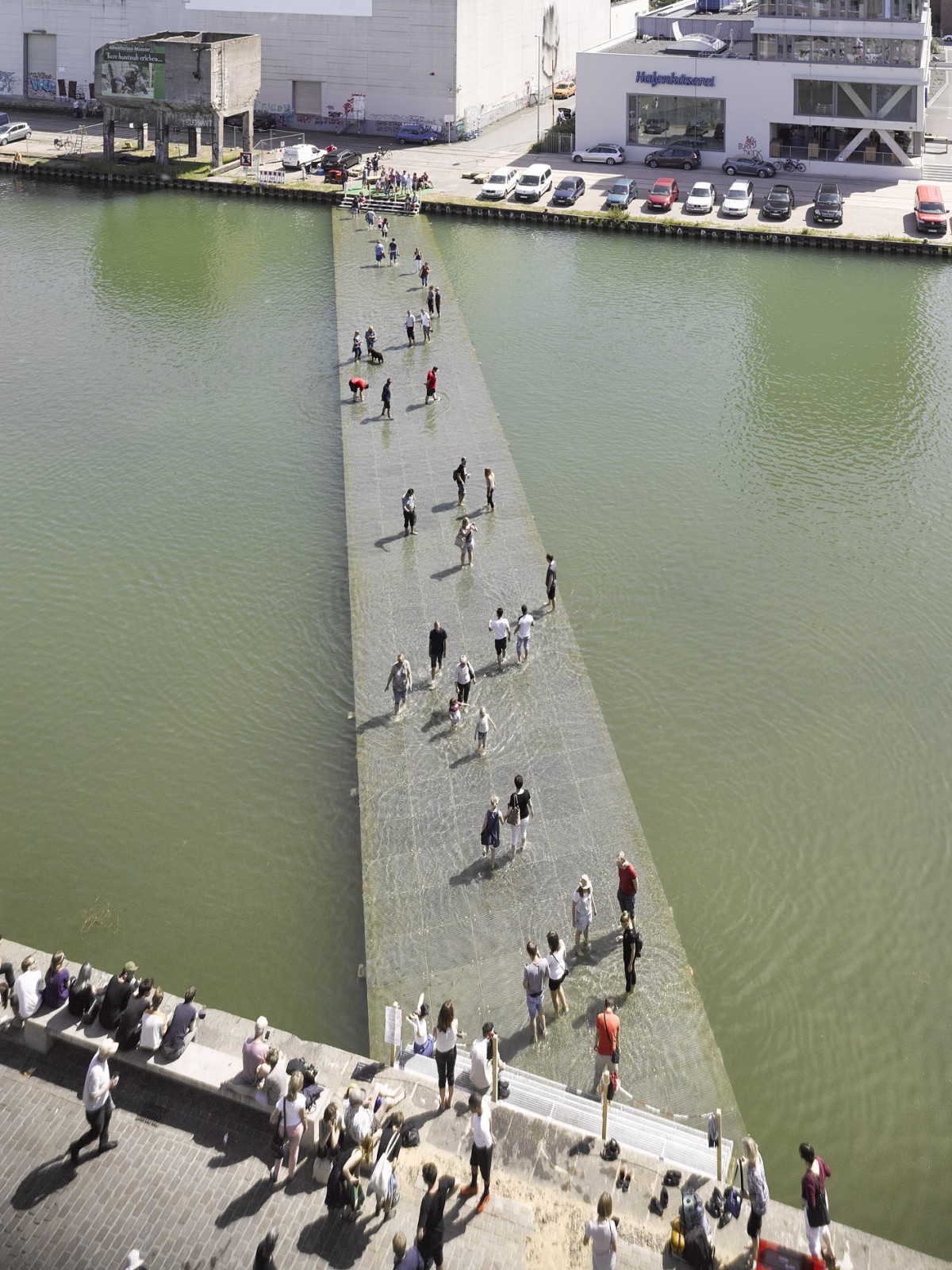This tall rectangular photograph offers a bird's eye view of a unique underwater pedestrian bridge, stretching diagonally across a murky, greenish-gray waterway from the bottom right to the top left. The gray, tile-constructed bridge is submerged just enough for people to enjoy a refreshing walk with their feet in the shallow water. In the foreground, a gray brick pier with white benches is visible, where people are standing, sitting, and taking off their shoes before venturing onto the bridge. This area transitions into a carefully maintained shoreline with additional benches and pedestrian walkways. Across the waterway, there is a parking lot and various modern structures including an office building and a factory-like establishment. Cars are parked lining the road that faces toward the camera. The photograph, measuring five inches wide by eight inches tall, captures a moment of communal relaxation and interaction, with people leisurely walking back and forth on the submerged bridge, enjoying the novel experience and the sense of community it fosters.